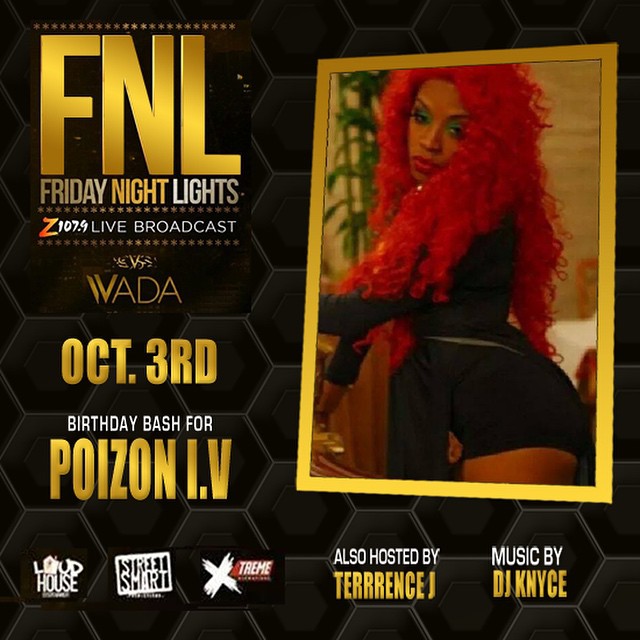**FNL Friday Night Lights Poster Ad**

**Join Z107.9 for a Live Broadcast!**

*Date:* October 3rd

*Event:* Birthday Bash for Poison Ivy (P-O-I-Z-O-N-I.V)

*Featuring:*
- Special host Terrence J
- Music by DJ KNYCE

*Details:*
- Eye-catching ad with a black background, hexagon pattern, and striking gold text.
- Large gold letters: **FNL**
- Underneath: **Friday Night Lights**, **Z107.9 Live Broadcast**
- In a gold-trimmed box on the right, a photo of a stunning black woman with bright red, curly hair, wearing a black romper and blue eyeshadow, leaning against a couch.
- Background includes a plant and brown window shades.
- Bottom logos: **Loud House**, **Street Smart**, **Xtreme** (twice for emphasis).

Don’t miss out on the party of the year, live on Z107.9!